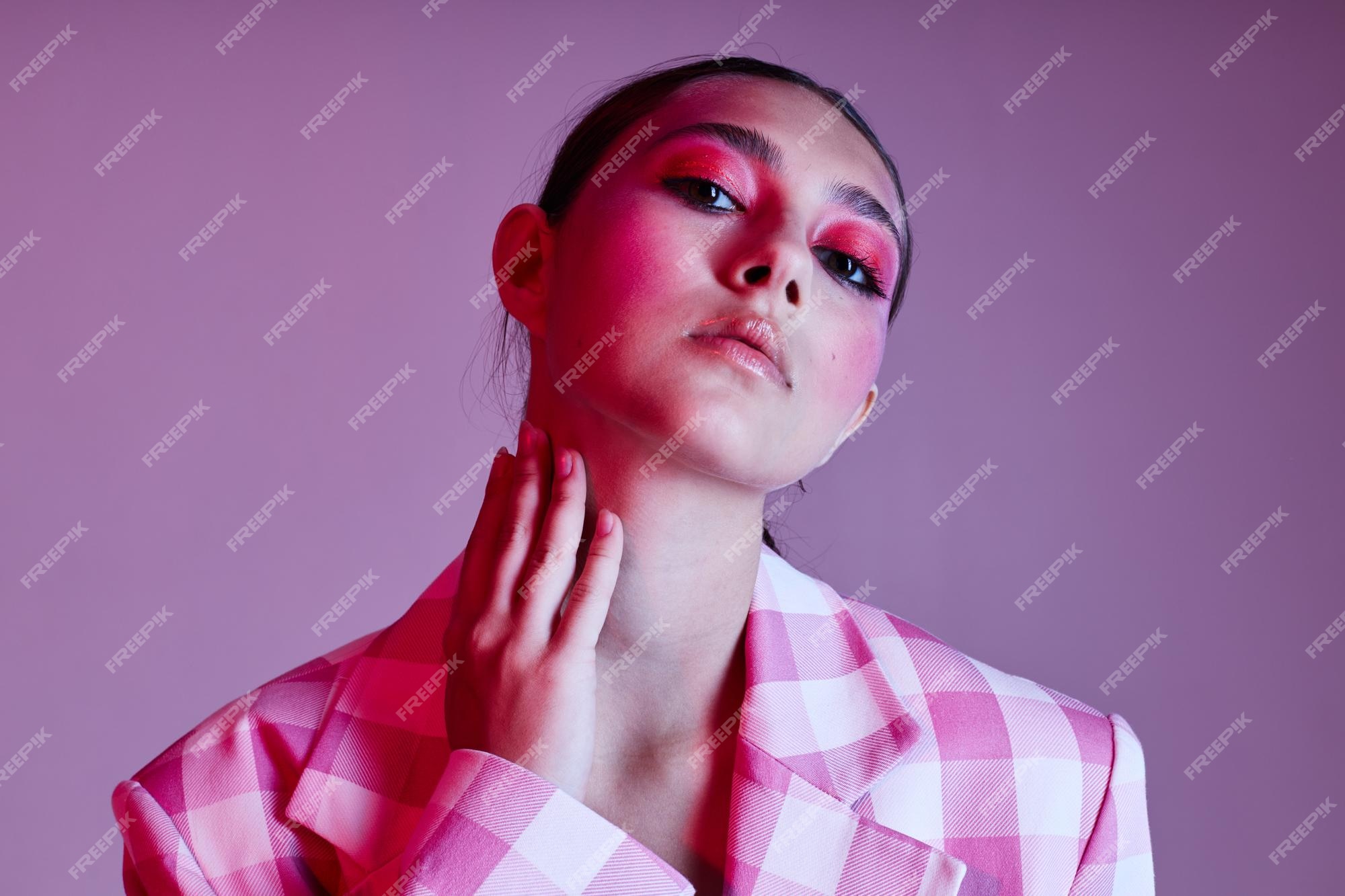This is a detailed photograph of a young woman in her 20s set against a pinkish-purple background, watermarked with the text "Freepik." She has captivating black hair, styled loosely behind her ears with a few strands cascading down her back. Her brown eyes are accentuated with pink eyeshadow and mascara, while she wears pink lipstick, enhancing her elegant appearance. The woman is wearing a pink and white plaid blazer with long sleeves, and her fingernails are painted pink. She is posing with her right hand gently caressing the side of her neck, her head tilted slightly back and to the left, creating a graceful yet introspective expression as she looks directly into the camera.